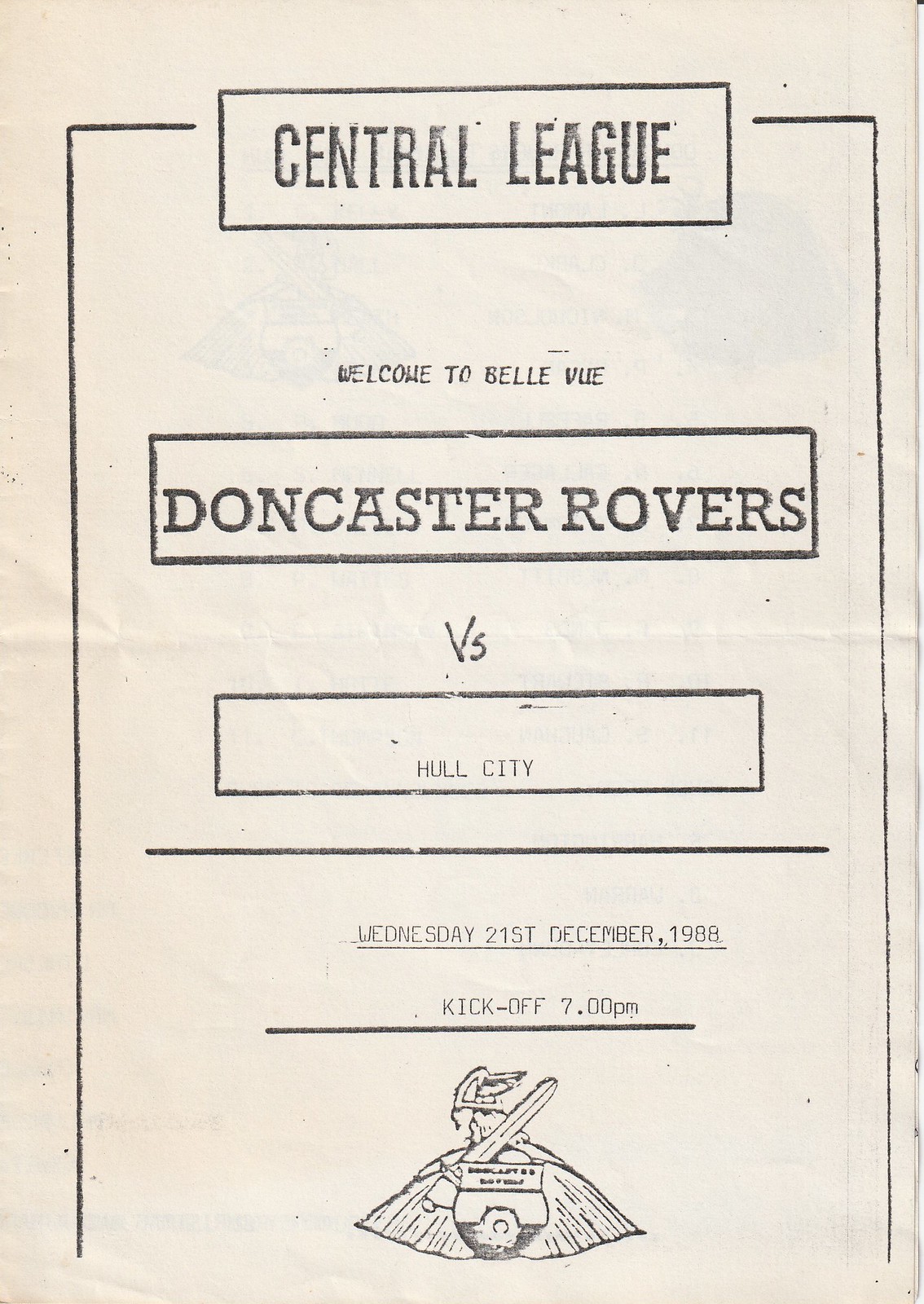This image shows an aged, off-white sheet of paper, possibly a pamphlet or program, with black text and rudimentary print, likely created using a typewriter. Encasing the entire document is a thick black border. At the top, a horizontal black rectangle prominently displays "CENTRAL LEAGUE" in large, bold, black capital letters. Beneath this, in smaller black capital letters, is the text "WELCOME TO BELLEVUE."

Further down, there is another black rectangle containing the larger text "DONCASTER ROVERS," followed by the word "VS" in smaller font. Below that, within another black box, the name "HULL CITY" appears in small, typewriter-like font. A divider line separates this section from the subsequent details, which include the underlined date "Wednesday, 21st December 1988," followed by the text "Kickoff 7 PM."

At the very bottom, centrally positioned, is the Doncaster Rovers logo, which depicts a Viking warrior. This somewhat crude logo features a Viking in a winged helmet, holding a sword diagonally, with a shield emblem in front of him, and appears to be viewed from a side profile, looking to the left. Observers might see additional indistinct details within the logo.